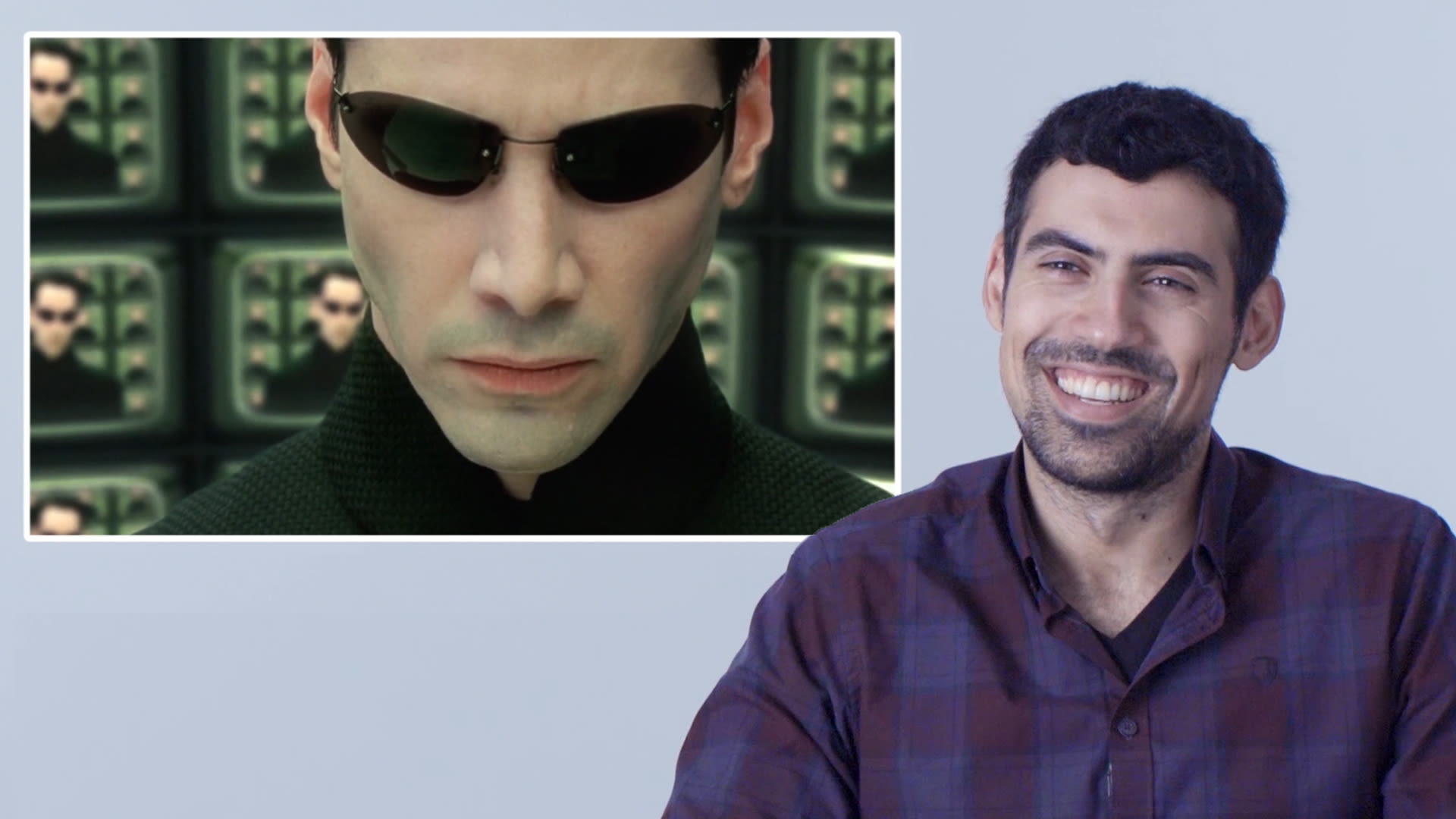The image features two main subjects. On the left-hand upper corner, there is a close-up of a man with black sunglasses, a black shirt, and a grimace on his face. Surrounding this man, there are multiple screens displaying the same exact image of him, arranged in rows where some are partially blocked. This figure appears to be a depiction of Keanu Reeves from *The Matrix*, featuring his iconic look with a bluish-gray and black background.

On the right side of the image, there is another man with dark brown hair, wearing a blue and maroon checkered, long-sleeved button-down shirt over a black V-neck t-shirt. He has a scruffy beard and a mustache, and a huge smile on his face, seemingly laughing. The man appears to be between 25 to 35 years old and looks like he might be reminiscing about a role he played, possibly because of the resemblance to the character on the left.